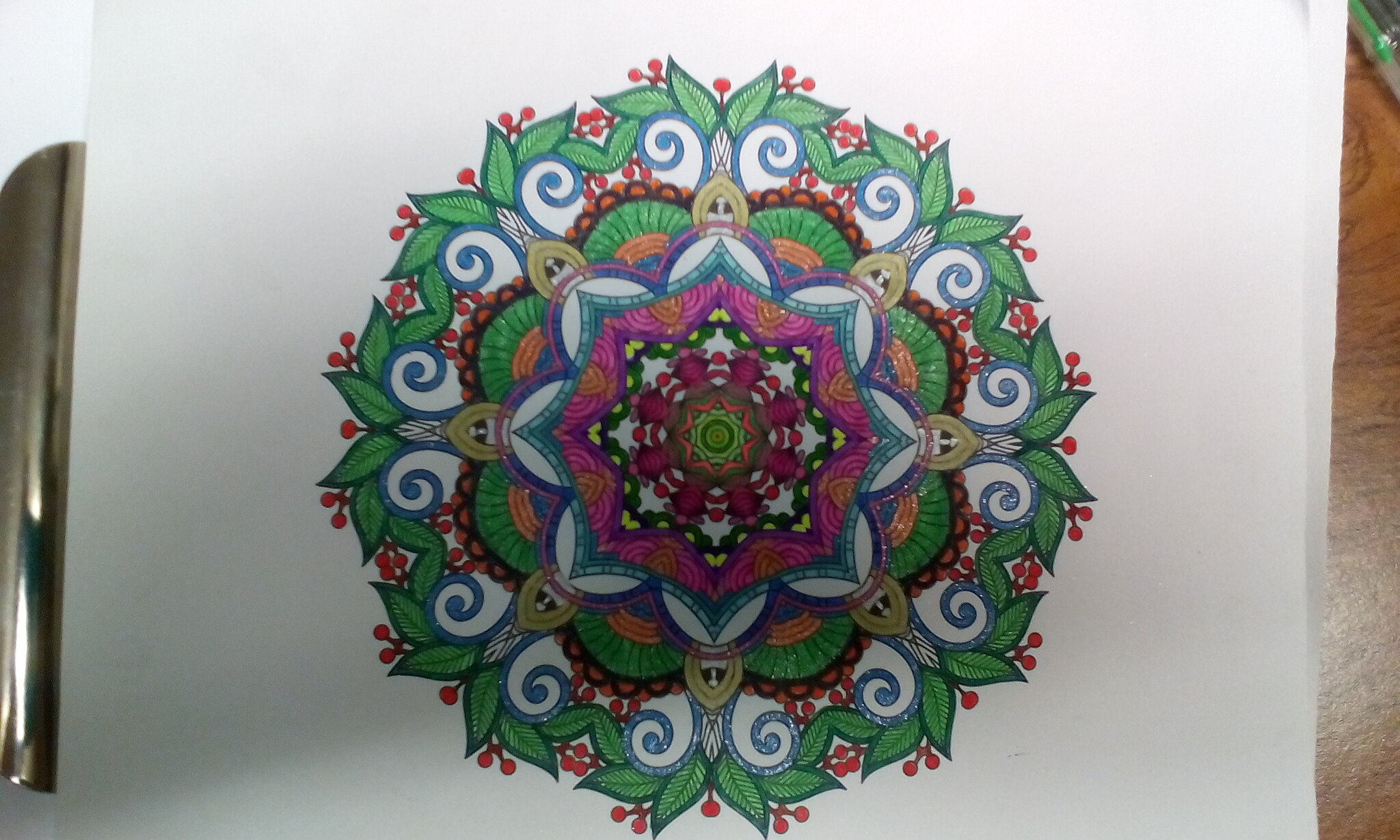A hand-drawn artwork on a plain piece of white paper captures a captivating, ornate design. The central focus is an intricate, astral-religious themed motif. Surrounding the center is a wreath-like formation of green leaves, radiating outwards. Encompassing this ring are whitish-blue, wave-like or tentacle-esque extensions that add a celestial touch. At the core of the design is a distinctive, purplish hexagonal shape, encasing another concentric circle. Inside this secondary circle lies a green hexagon with eight points, each capped with a small green circle. Scattered around the composition are red, berry-like embellishments that provide a pop of color. The artwork is set on a plain piece of white paper, slightly revealing the brown surface of a table underneath and held in place by a silver clipboard clip. The use of various colors suggests it was created with colored pencils or markers, lending a vibrant, multi-dimensional appearance to the piece.